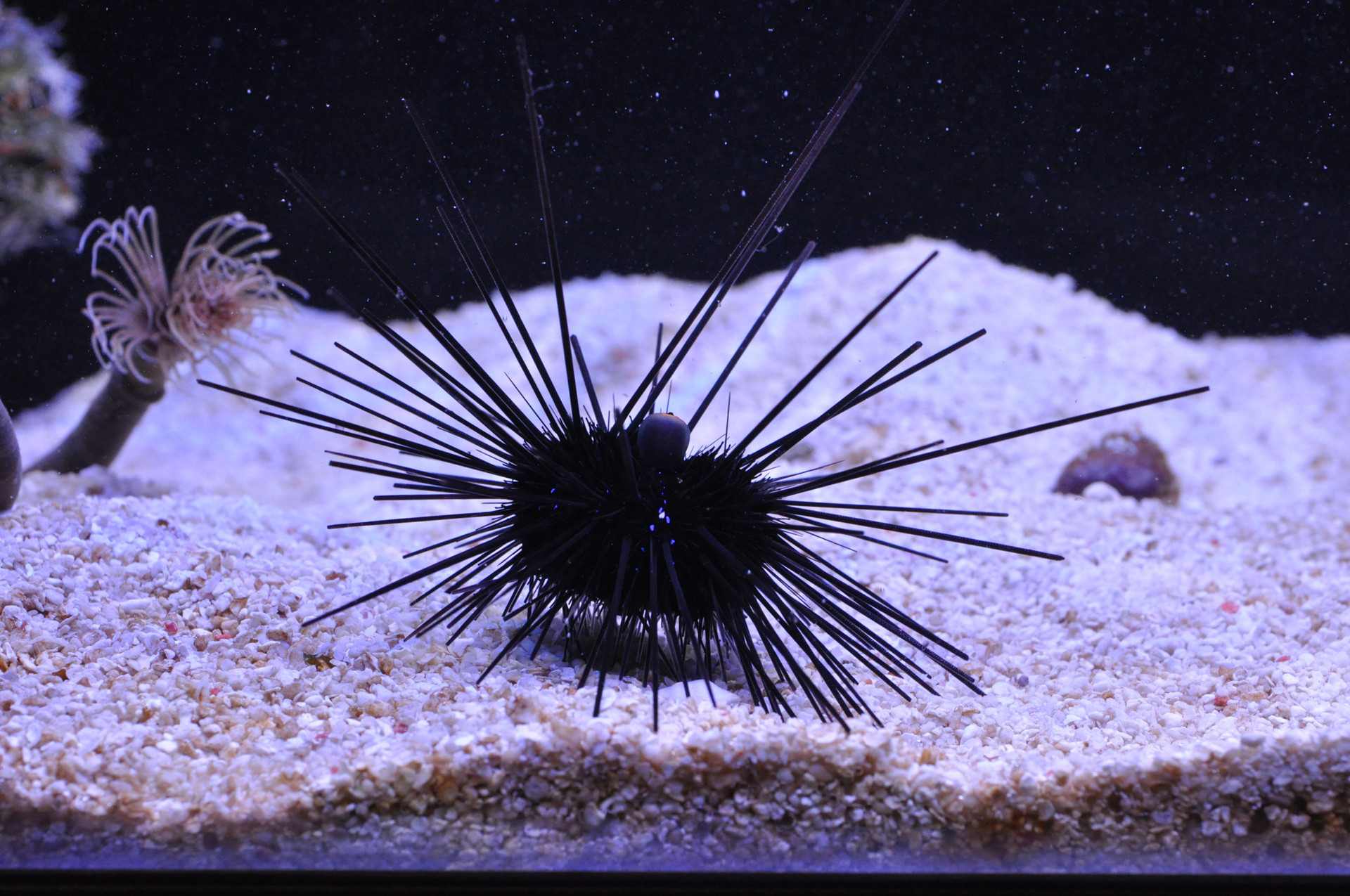This detailed color photograph, likely taken in an aquarium, captures an underwater scene featuring a black sea urchin. The sea urchin, resembling a big, spiky black ball or hairy blob, is adorned with dozens of long, thin, sharp spines radiating in all directions. The spines are notably longer on the top, left, and right than those closer to the sandy base. The urchin is situated on a gravel bed composed of light-colored particles in hues of beige, white, and light violet.

To the left of the sea urchin is an intriguing aquatic plant that stands out with its light brown stem and delicate branches, somewhat resembling a miniature palm tree with pinkish and beige feelers at the top. Additionally, a small sea creature with numerous tentacles is positioned near this plant. On the right, there's a prominent brown rock, contributing to the diverse textural landscape. The background consists of dark water interspersed with small, white floating specks and rising mounds of gravel or sand, adding depth to this captivating underwater tableau.